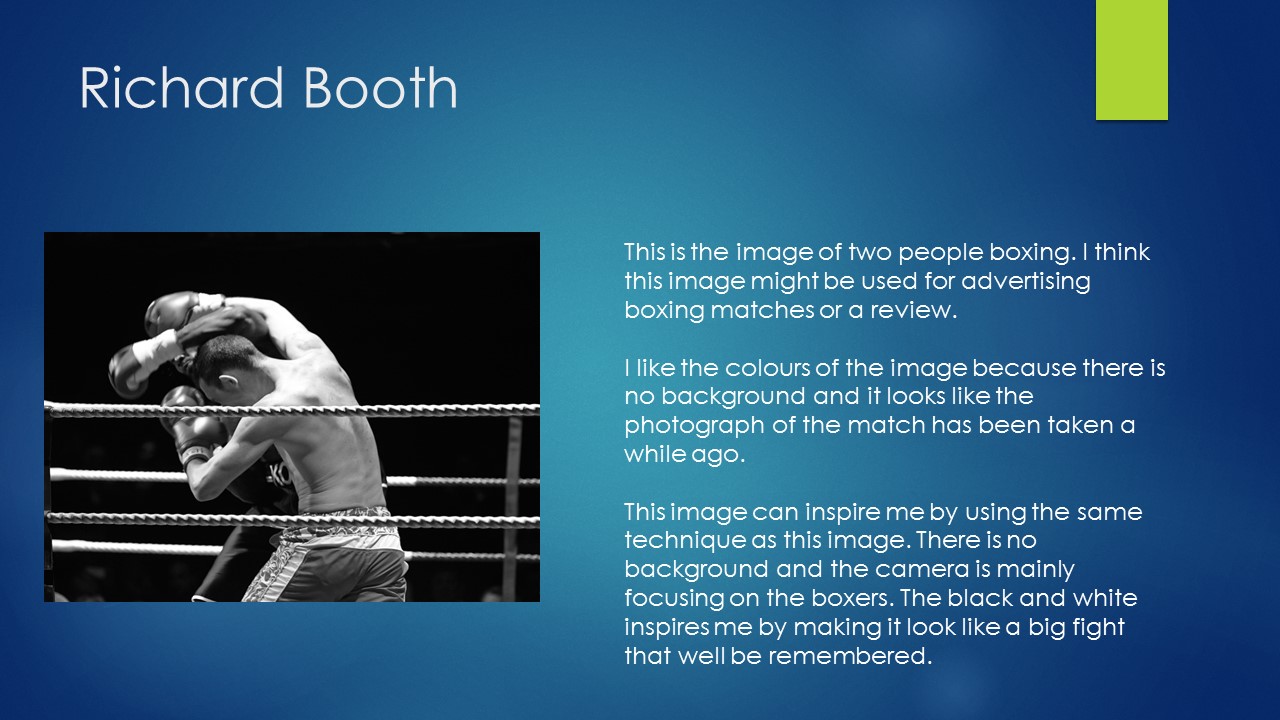The image is a PowerPoint slide featuring a blue gradient background with a neon green bookmark-style marking at the top. The title "Richard Booth" is prominently displayed in white sans-serif font at the top left corner. Below the title, there is a black-and-white photograph of two men boxing in a ring, both wearing boxing shorts, shirts off, and gloved hands raised. The boxing ring ropes are visible, adding context to the scene. Across the right side of the slide, there are approximately three paragraphs of white text that describe how the image is inspiring to the author. The text also speculates that Richard Booth might be the photographer, as the techniques and vintage look of the photograph are admired. This slide may be used for advertising boxing matches or could be part of a review, emphasizing the timeless and memorable nature of the fight captured in the image.